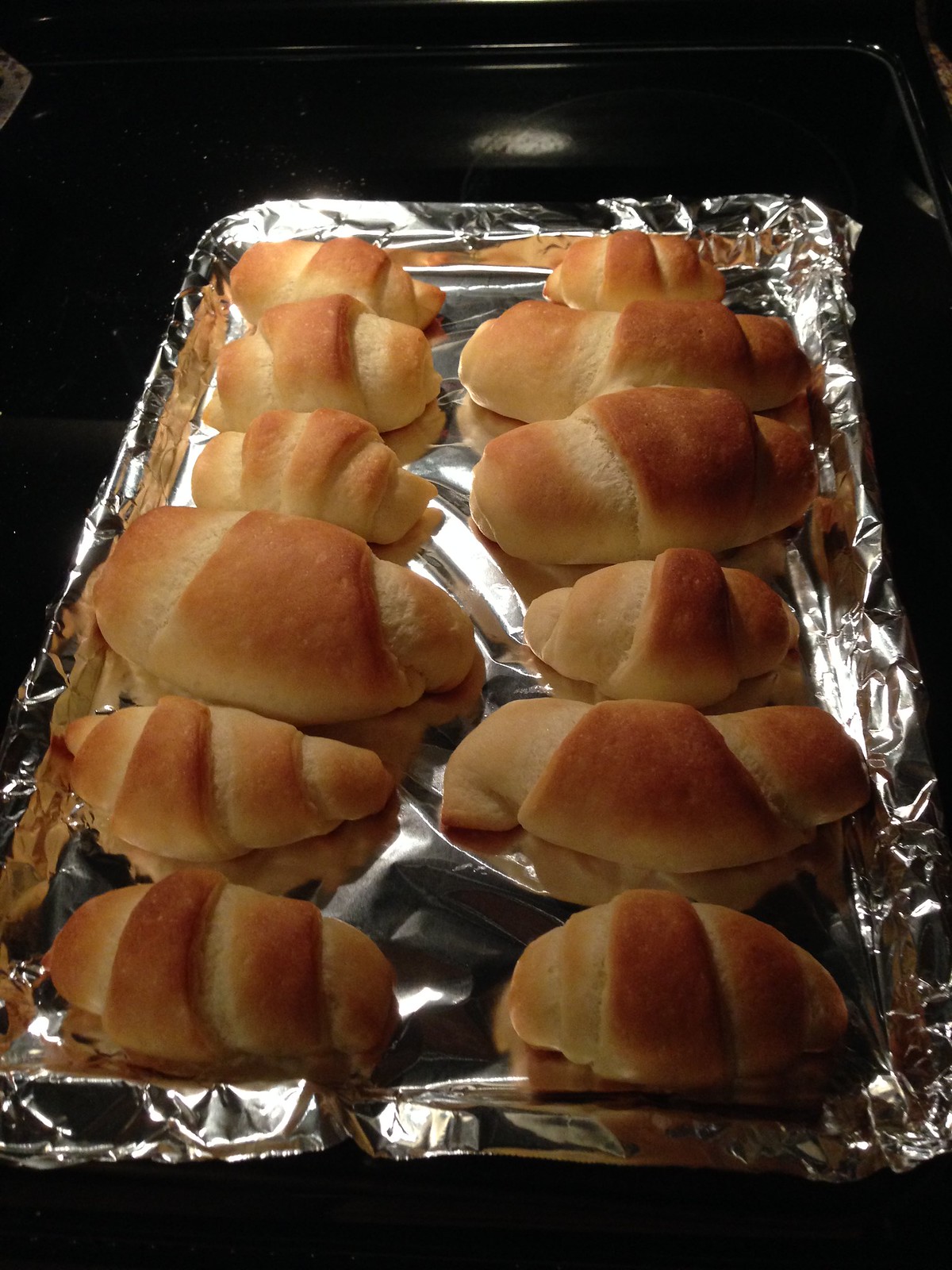In this image, we see a freshly baked tray of crescent rolls arranged on a sheet of aluminum foil that completely covers the cooking tray beneath. There are 12 crescent rolls, neatly aligned in two rows with six columns each. They vary in size and shape; some are small and puffy, some are larger and more elongated, and others are medium-sized. The rolls are perfectly golden brown, although some show slight scarring on the sides, adding to their rustic charm. The aluminum foil appears to be neatly wrapped around the tray, which sits on a shiny black surface that resembles the inside of an oven. These plain crescent rolls, with their enticing golden crust, seem ready to be enjoyed fresh out of the oven.